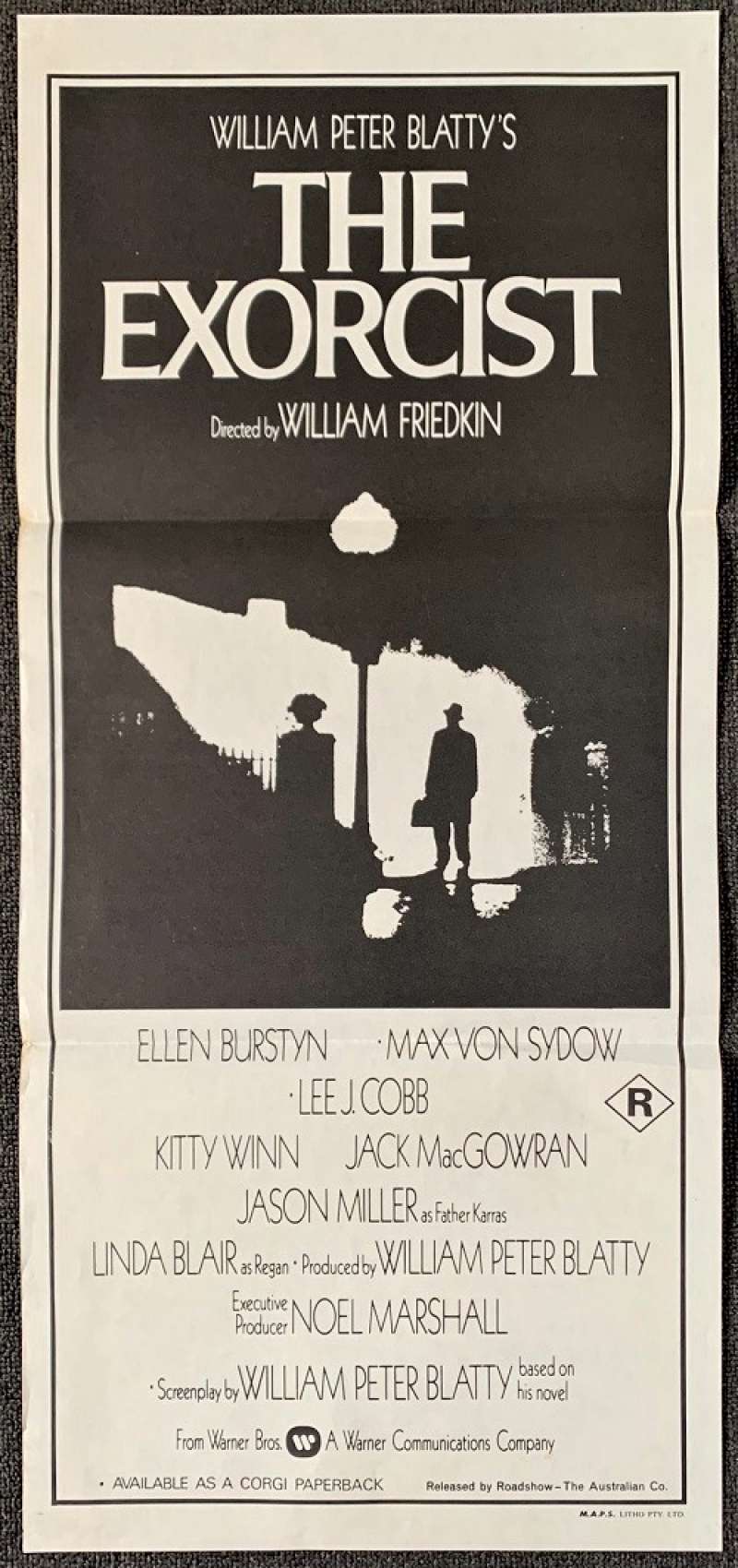This framed poster, likely from the 1970s, is a narrow, tall movie poster for "The Exorcist," featuring a plain black and white design. The top of the poster showcases the iconic image of a priest arriving at a house, his silhouette backlit by a street lamp, capturing a scene from the film. The text at the top reads "William Peter Blatty's The Exorcist, directed by William Friedkin," all set against a black rectangle background. Below this, a white text box lists the cast: Ellen Burstyn, Max von Sydow, Lee J. Cobb, Kitty Winn, Jack McGowran, Jason Miller as Father Karras, and Linda Blair as Regan.

The poster is bordered with a black frame, and the area around the poster includes color elements—black, pink, and white borders. Additional details include the Warner Brothers logo and the rating (R). The poster appears to be an original period piece with minor yellowing and fold marks, adding to its vintage charm.